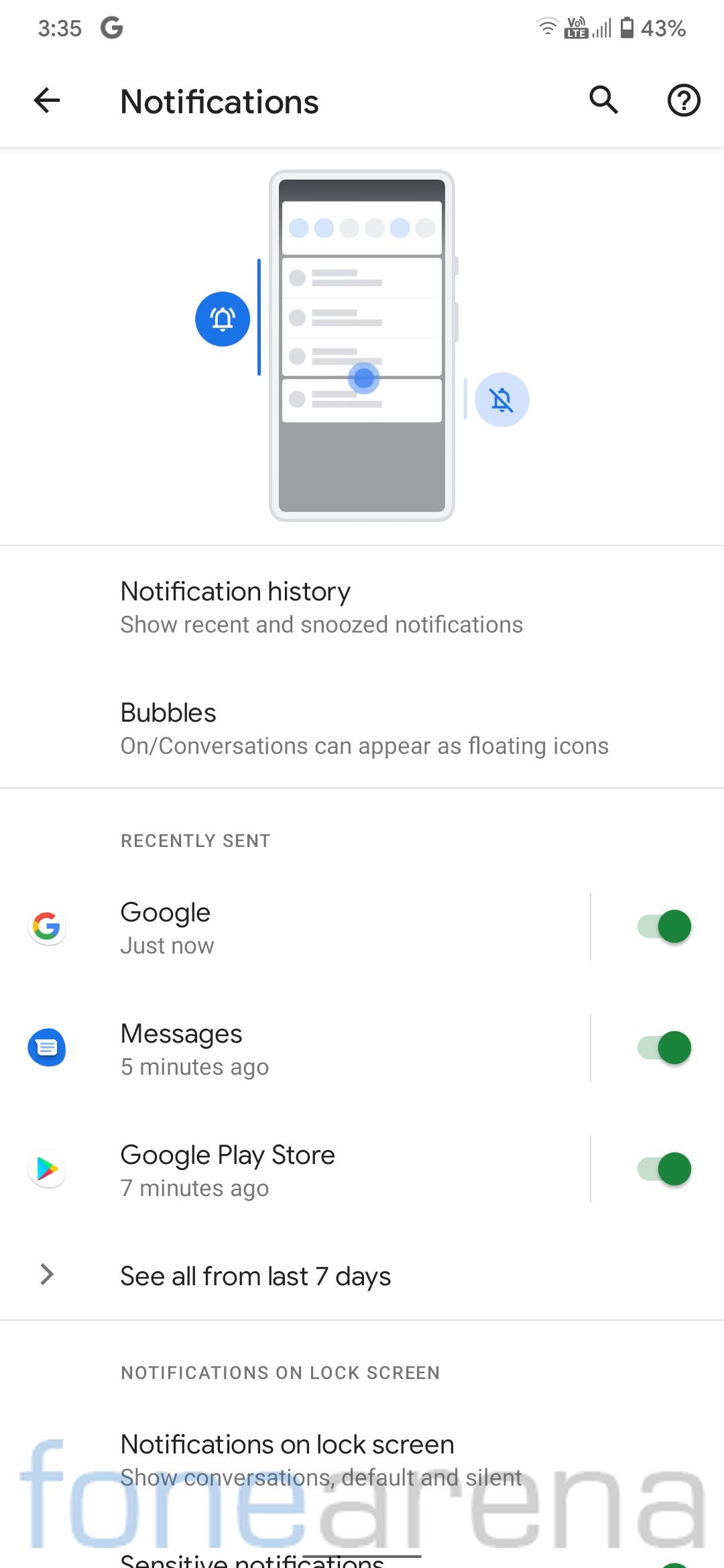This image showcases the notification settings interface of a smartphone, likely focusing on a mail application. The section opens with a title that reads "Notifications" at the top. A graphic depicting a vibrating phone is prominently displayed, symbolizing that notifications are active. Below the image, in the notification history, several recent alerts are listed: one from "Google" labeled "Just now," a "Messages" notification from 5 minutes ago, and an alert from the "Google Play Store" received 7 minutes ago. A link to "See all from 7 days ago" is also present, offering access to an extended notification history. Further down, the settings for "Notifications on lock screen" and "Sensitive notifications" are mentioned, emphasizing privacy and visibility options. The presence of multiple iconography and text entries underscores the detailed configurability of the app's notification system.